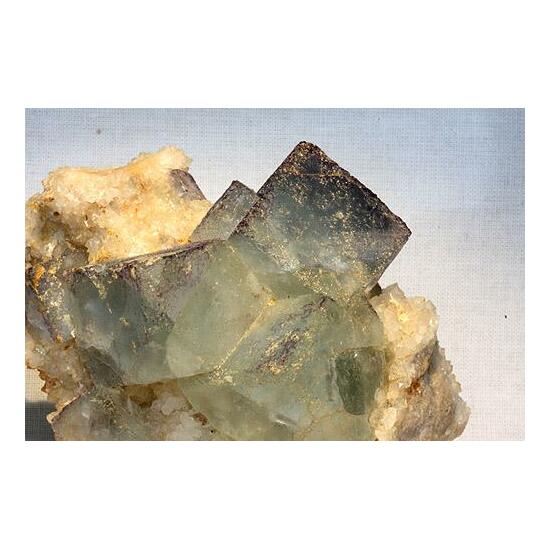This image showcases a very close-up view of a sizable, unpolished mineral formation, likely a geode. The central feature is a cubical rock structure comprising multiple interlocking sections, giving it a blocky and complex appearance. The mineral is predominantly yellow with accents of brown, black, and green. Specks of dust are visible on its reflective surfaces, emphasizing its raw state. Positioned on the left side and occupying about 60 to 70 percent of the image, the formation is still partially embedded in its surrounding earth, which consists of white and tan hues. The background of the image features a gradient that transitions smoothly from gray at the top to blue in the middle and then to white at the bottom, providing a neutral contrast that highlights the intricate details of the mineral.